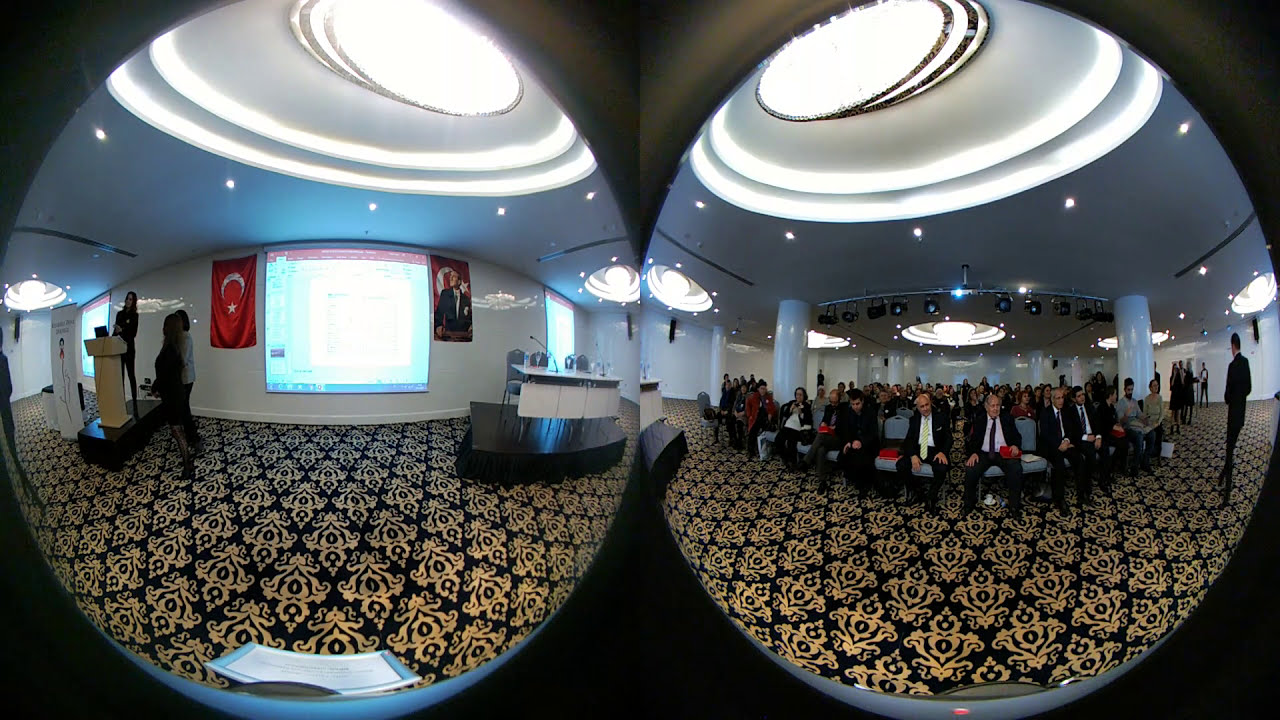The image presents a double fisheye view of an expansive, carpeted conference room. The fisheye effect creates two circular images: the right image captures rows of fold-out chairs with cushions, nearly filled as far as the eye can see with people dressed in business attire, predominantly men in suits. The left image mirrors the same room but from a reverse angle, focusing on what the audience is observing. This view includes a pull-down screen, a podium to the left, and a desk on a raised surface to the right. Three women are positioned to the left of the screen, one of whom stands behind the podium. The room's black carpet features diamond-shaped gold symbols, and the ceiling, with a bluish tint, is adorned with globe lighting. There are also two prominent columns in the middle of the room, adding to the sophisticated ambiance of the space.